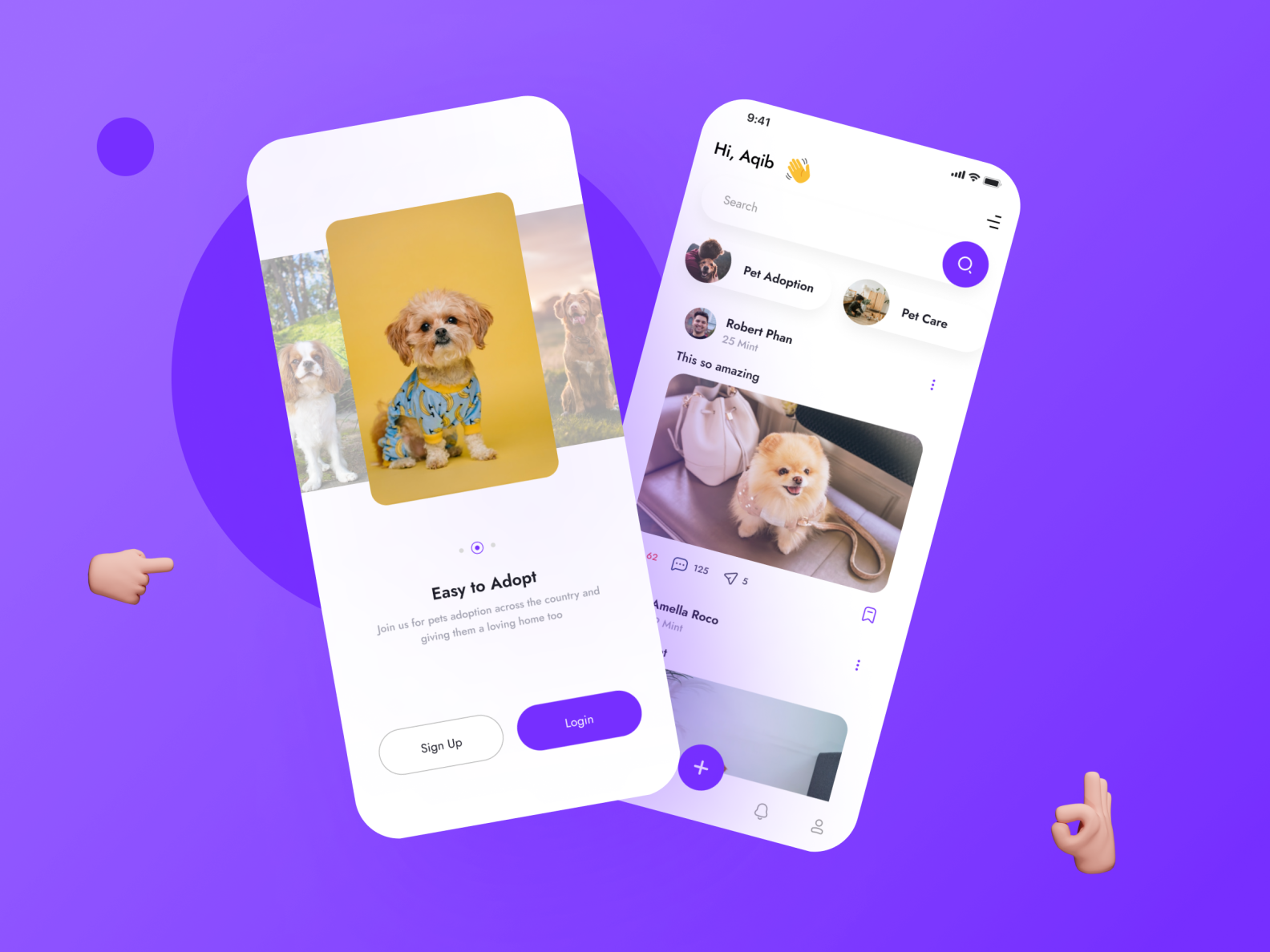This image gallery promotes a national pet adoption campaign, emphasizing the ease and importance of adopting dogs, and inviting viewers to join the effort in giving these animals a loving home. The first image highlights four different dog breeds available for adoption, including a chihuahua, which is well-known and cherished as a pet breed. The gallery interface displays several on-screen elements: a sign-up button, a log-in button, a notification bell, and user account buttons on the top navigation bar. Additionally, the interface shows a fully charged battery, strong Wi-Fi signal, and a 3-hour stay logged in, indicating an active and engaged user experience. The captions celebrate the amazing opportunity to adopt and care for these pets, emphasizing the user-friendly platform designed to facilitate the adoption process. Each image is thoughtfully accompanied by relevant information to encourage and assist potential pet owners in making a difference.